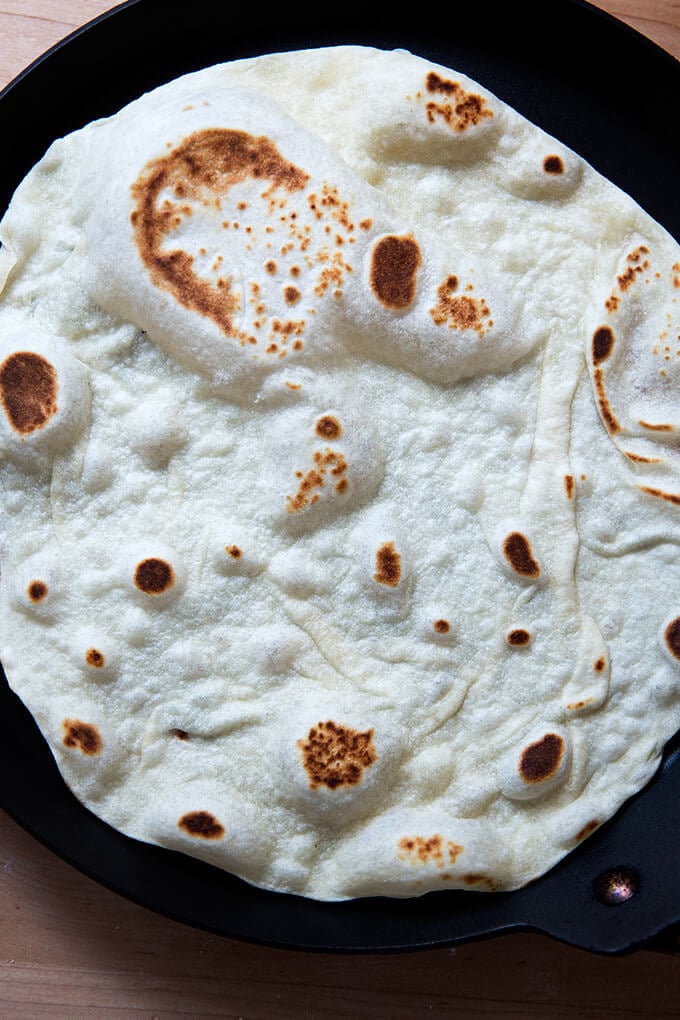This detailed indoor photograph, shot from above using artificial lighting, features a homemade fried flour tortilla sitting in a black cast-iron skillet on a light wooden table. The image is vertically rectangular with faint hints of the wooden table and rounded black edges of the skillet visible in the corners. The tortilla, showcasing an off-white hue with distinctive browning and bubbling, appears cooked to perfection, characterized by a variety of scorch marks ranging from dark to light brown. These spots and bubbles suggest it was freshly fried in the pan, creating a textured surface reminiscent of the moon. The tortilla isn't quite the full diameter of the skillet, leaving about an inch of space around the edges, and the photograph's detailed capture makes it ideal for illustrating a homemade tortilla recipe, visually guiding viewers on the desired doneness and texture.